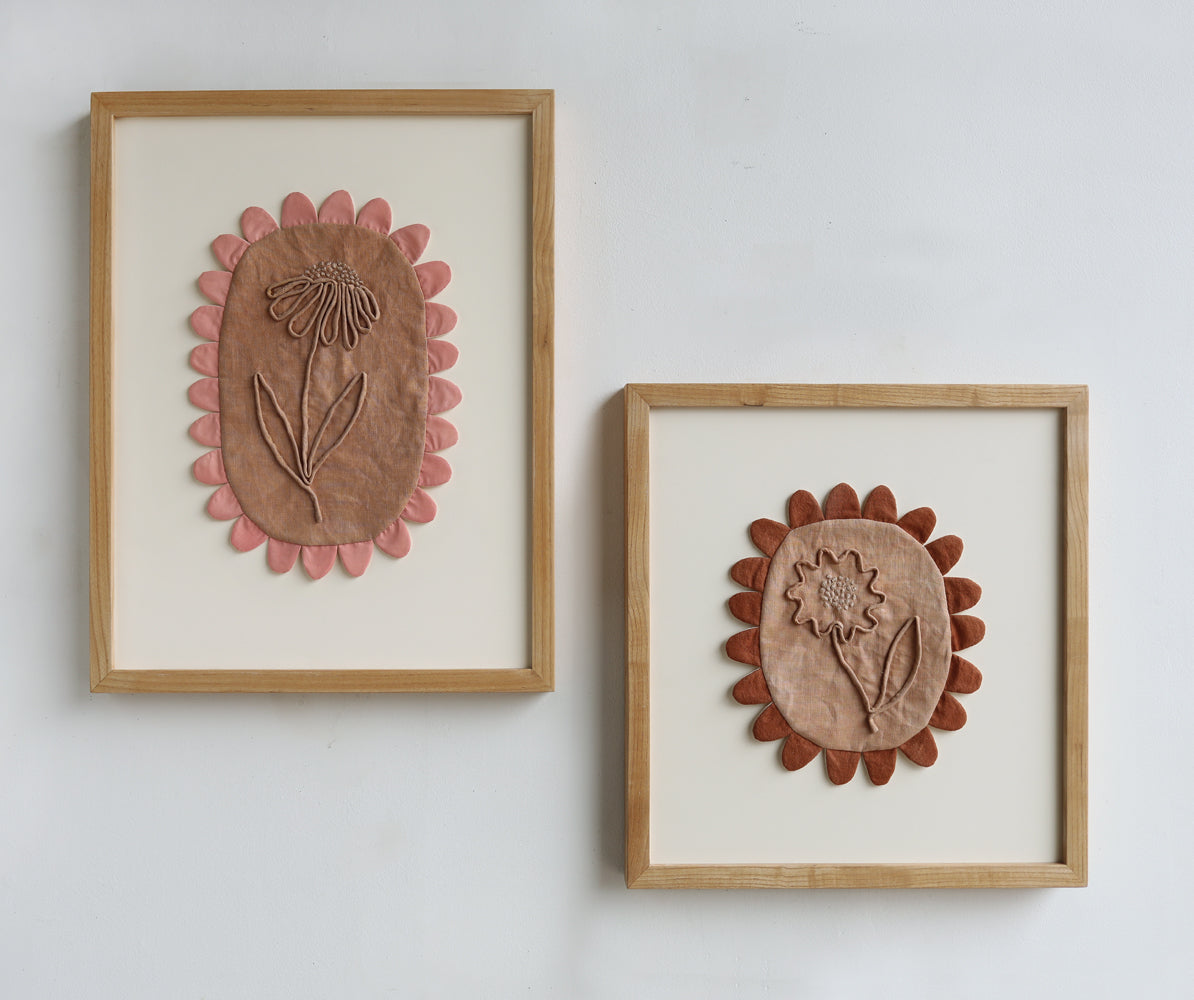The image is a color photograph depicting two framed textile artworks hanging side by side on a white wall. Both frames are made of light brown wood and the artworks are crafted from fabric, showing intricate embroidered floral designs. The artwork on the left is vertically oriented and set slightly higher than the square-format piece on the right. 

The left artwork features a suede-like, velvety light brown background with a centrally positioned flower that has long petals and French knot details at the top. The flower has a long stem with two leaves, one on either side, set against a white backdrop. The petals are a soft pink, contributing to the delicate appearance of the piece.

The right artwork, hanging lower and in a square format, showcases a roundish floral design with a lighter center compared to the left piece. The petals, in shades of dark brick red, encircle the central elliptical flower, which seems to be outlined with macrame or rope, incorporating white dots in the middle. The background is similar to the left piece but presents a slightly darker hue to the flowers.

The artwork style combines textile 3D sculptural effects with photographic representational realism, creating a rustic yet elegant aesthetic. The frames' simple design and the harmonious colors of pink, orange, and beige, enhanced by soft grayish-blue shadows, draw attention solely to the embroidered flowers without any extraneous elements.